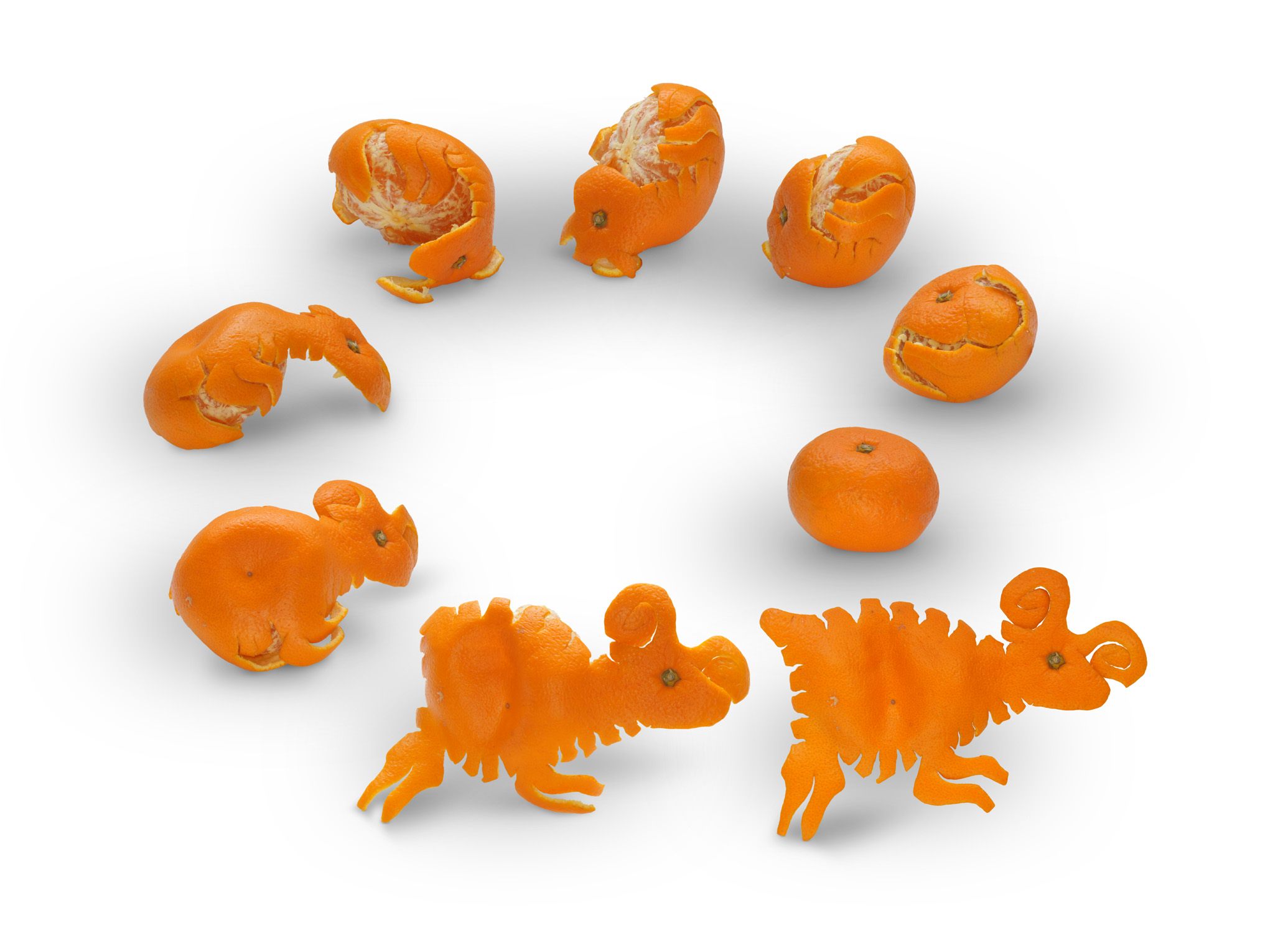The image depicts a captivating sequence involving a mandarin or tangerine, presented as a visual narrative in a counter-clockwise circular arrangement. At the center lies a whole, unpeeled mandarin. As you follow the sequence, the mandarin gradually transforms through various stages of peeling and evolves into a visually engaging form. Initially, each stage reveals more of the peel being lifted until the peel completely separates from the fruit. Progressively, the peeled sections artfully morph into the shape of a ram or antelope, complete with curled antlers and four legs, using the mandarin's stem as the eyes. This creative depiction culminates in a sophisticated sculpture where the peel alone stands as a detailed representation of the animal, demonstrating a remarkable evolution from a simple fruit to an intricate piece of art.